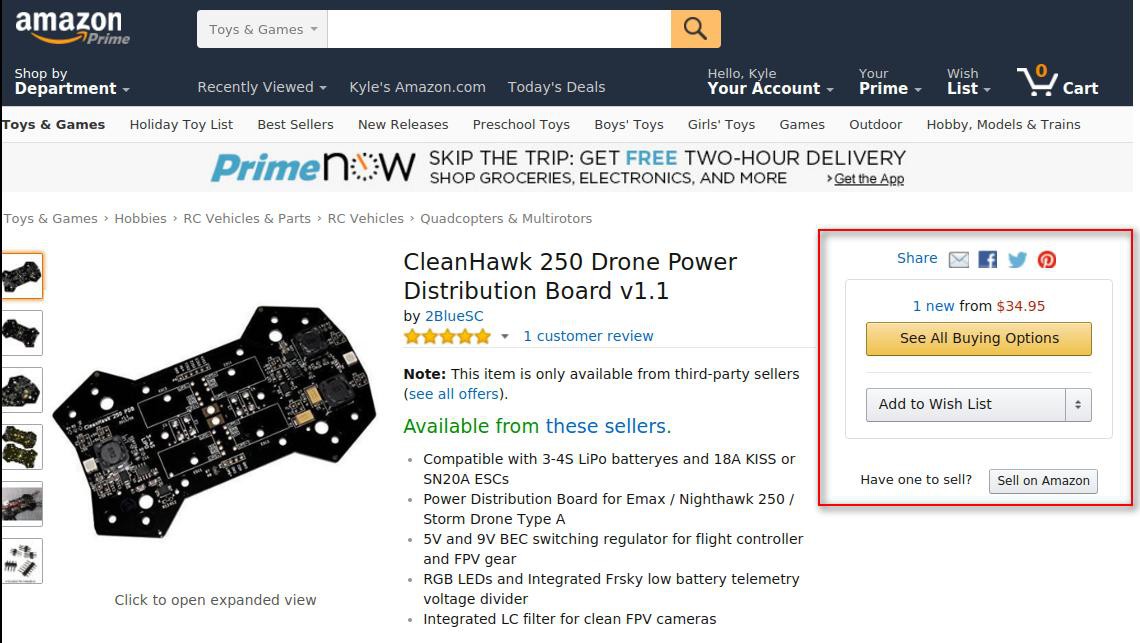**Detailed Description of the Amazon Webpage Image:**

The image depicts an Amazon webpage interface showcasing various features and options available to the user. At the top of the page, prominently displayed, is the "Amazon Prime" banner. Adjacent to it is a search box pre-set to filter results within the "Toys & Games" category. The navigation bar includes several options: "Shop by Department," "Recently Viewed," "Kyle's Amazon.com," and "Today's Deals." Beneath these options, the page greets the user with "Hello, Kyle," alongside links to "Your Account," "Your Prime," "Wishlist," and a shopping cart icon indicating zero items.

Further down, a list of subcategories within "Toys & Games" is visible, featuring options such as "Holiday Toy List," "Bestsellers," "New Releases," "Preschool Toys," "Boys Toys," "Girls Toys," "Games," "Outdoor," "Hobby Models," and "Trains."

Centrally located on the page is a product listing for the "CleanHawk 250 Drone Power Distribution Board V1.1." This product has received one customer review, boasting a five-star rating. The item is manufactured by 2BlueSC. The main product image showcases a black device with numerous components, suggesting its function in power distribution. In bold text, it is noted that this item is available only through third-party sellers, with a clickable link in blue text stating "available from these sellers."

The product description specifies its compatibility with "3, 4S LiPro batteries, and 18A KISS or SN20A ESCs." A highlighted box with a red border contains various interaction options, such as social media share icons, a "One new from $34.95" notice, a "See all buying options" button, and an "Add to Wishlist" feature. Additionally, there is a prompt that reads "Have one to sell? Sell on Amazon," encouraging users to list their items for sale.